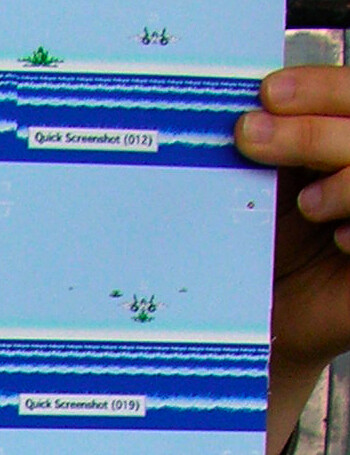A vertical rectangle photograph depicts a white left hand holding up a piece of paper against a light blue background. The upper part of the paper is solid light blue, featuring an indistinct image whose details are unclear. Below, a white line stretches across the paper, followed by a representation of green and some blue, resembling a tuft of grass or foliage. This is succeeded by several lines of computer-generated water in a darker blue, with evenly spaced white lines running horizontally across it.

Prominently positioned on this section of the paper is a white rectangle containing the text "Quick Screenshot (012)" in clear black print. Continuing downward, the paper transitions back to a large section of light blue. On the right side of this section is a small white square marked with a diamond shape. In the center of the light blue area below, there's a small, ambiguous image that appears to show two eyes, and possibly a nose and mouth, though it is not distinctly clear.

Further down, another white horizontal line appears, marking the transition back to the darker blue water motif with white lines. Once again, a white rectangle with the text "Quick Screenshot (0119)" is present, completing the lower section of the paper.